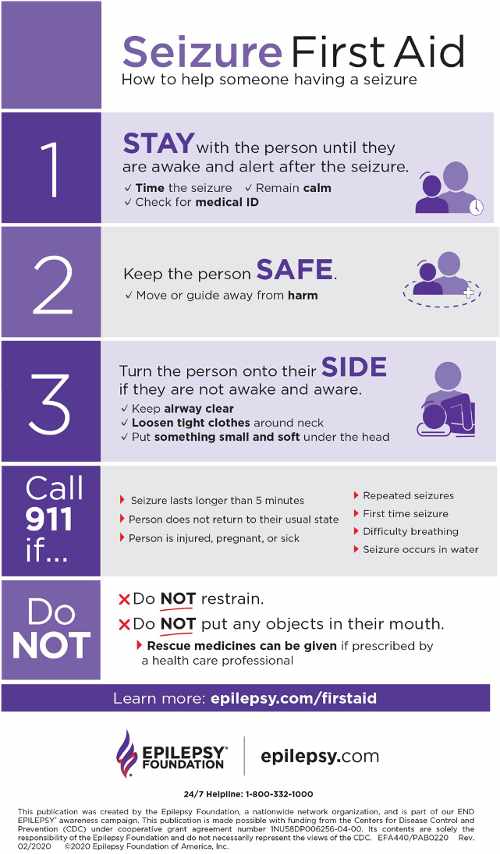This detailed instructional poster from the Epilepsy Foundation, titled "Seizure First Aid," features a clean white background with purple accents and provides crucial steps to assist someone experiencing a seizure. Prominently at the top, the title "Seizure First Aid" is displayed, with "Seizure" in bold purple and "First Aid" in bold black letters. Beneath this, the instructions begin with a smaller header: "How to Help Someone Having a Seizure."

The poster outlines a series of steps, each in a purple-themed design with a mix of text and small clip-art images. Step 1, titled "STAY" in dark purple capital letters, advises to "Stay with the person until they are awake and alert after a seizure." It further suggests timing the seizure, remaining calm, and checking for medical ID.

Step 2 commands, "KEEP THE PERSON SAFE," with "Safe" emphasized in bold capital purple letters. It instructs to move or guide the person away from harm.

Step 3 is in capital purple letters and emphasizes, "Turn the person onto their side if they are not awake and aware." Additional instructions include keeping the airway clear, loosening tight clothing around the neck, and placing something small and soft under the person's head.

Adjacent to these steps are smaller visual aids and beneath them, advice on when to call 911 — for instance, if the seizure lasts longer than five minutes, if the person does not return to their usual state, or if the person is injured, pregnant, or sick.

Lastly, the poster includes a “Do Not” section marked with red X’s to highlight what actions to avoid: do not restrain the person, do not put any objects in their mouth, and consider that rescue medicines can be given if prescribed by a healthcare professional.

At the bottom of the poster, the site reference "Learn more at epilepsy.com/firstaid" and the Epilepsy Foundation logo are present, anchoring the informative content with a trusted source for further learning.